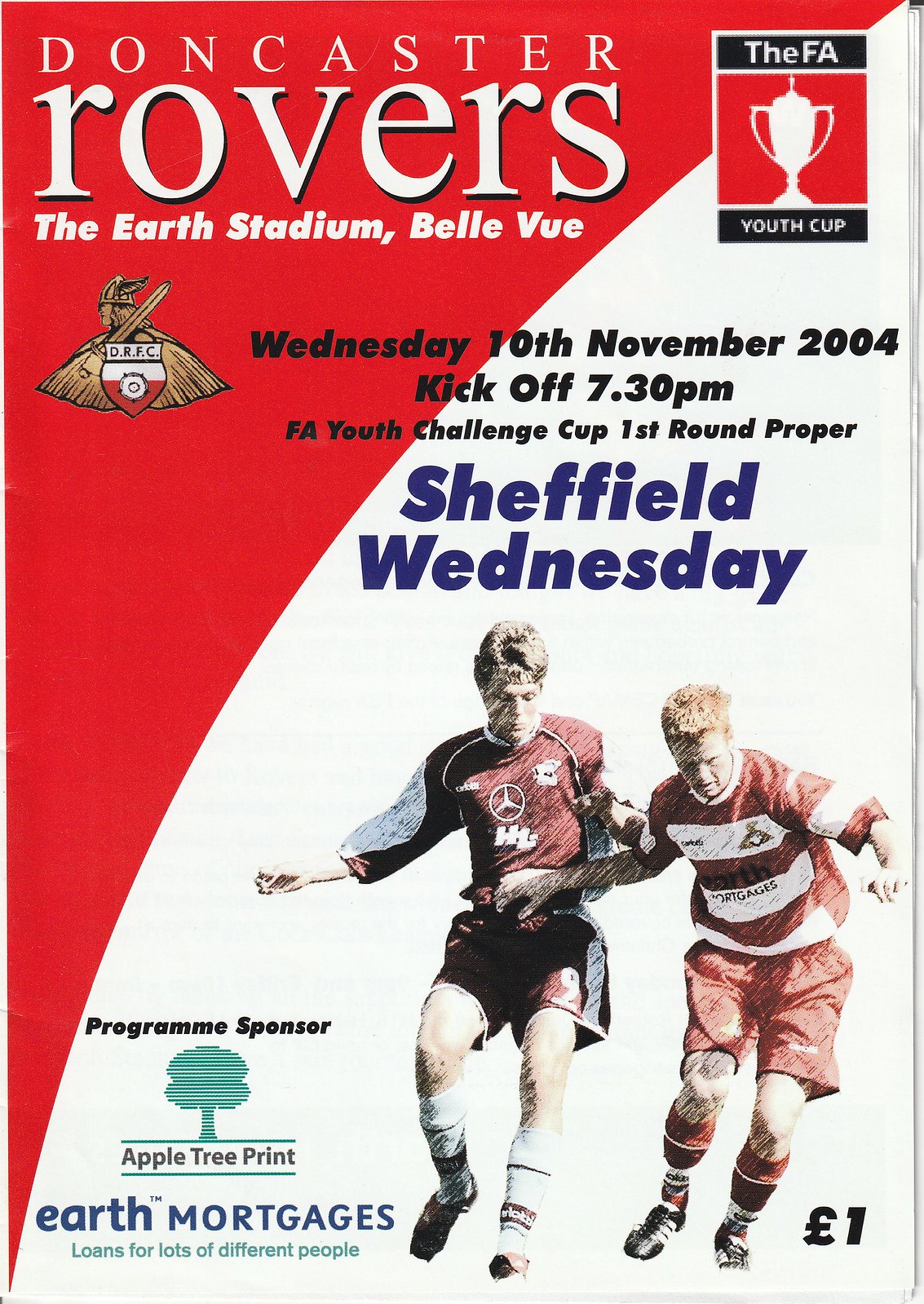The image displays the front cover of an English football club program for the Doncaster Rovers. The primary event detailed on the program is a match taking place at the Earth Stadium, Bellevue, on Wednesday, 10th November 2004, with a kickoff at 7:30 pm. This match marks the first round proper of the FA Youth Challenge Cup against Sheffield Wednesday.

At the top of the program cover, a banner runs diagonally from the top right to the lower left, displaying "Doncaster Rovers" and the Earth Stadium Bellevue details. Situated beneath this banner is a team logo featuring a Viking helmet with wings and a sword, marked "DRFC." Adjacent to the banner, on the upper right side, is the FA Youth Cup logo, which includes an image of a trophy.

In the central part of the cover, two soccer players from different teams are depicted: one dressed in a maroon top with black shorts, and the other in a red top with red shorts. They are against a white background, with a red area above them, separated by an arc.

The program also prominently features the sponsors at the bottom left corner: Apple Tree Print and Earth Mortgages, which offer loans for various people. Additionally, the program's price is marked as one pound.

Overall, the detailed visual and informational elements collectively emphasize the significance of the event, the competing teams, and the support from the sponsors.